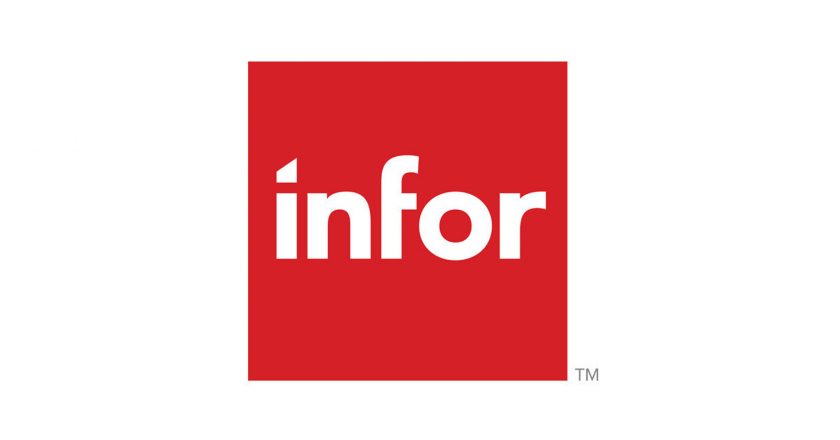This simple yet eye-catching image features a square-shaped graphic design against a clean white background. Dominating the lower right-hand corner, this solid red square, approximately 2 inches by 2 inches, displays the word "infor" (I-N-F-O-R) in bold, white, stylized lowercase letters. Notably, the dot above the "i" is an irregular parallelogram, slanted to be higher on the right side. Just outside the red square in the lower right corner, in very small, light gray capital letters, are the initials "TM". This minimalist design highlights the modern use of typography and color to convey a succinct message.